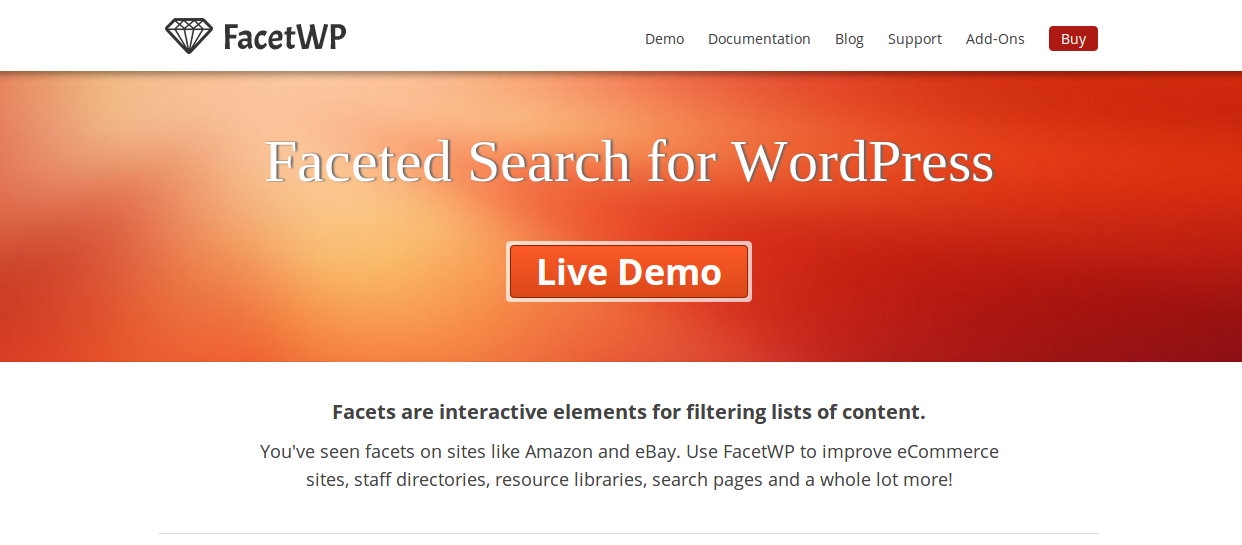The image features a clean and professional layout, with a white border at the top. At the center, there is a digital drawing of a diamond, accompanied by the text "Facet WP." To the right of this image, there are navigational links labeled "Demo," "Documentation," "Blog," "Support," and "Add-ons." Below these links, there is a prominent red button labeled "Buy."

Directly underneath, another red rectangular box displays the message "Faceted Search for WordPress," emphasizing the primary theme of the page. Below this, there is another box with a white border that invites users to explore a "Live Demo."

Further down, descriptive text explains the utility of facets: "Facets are interactive elements for filtering lists of content." It continues to elaborate on the versatility of the Facet WP plugin by noting, "You've seen facets on sites like Amazon and eBay. Use Facet WP to improve e-commerce sites, staff directories, resource libraries, search pages, and a whole lot more." A subtle light gray line extends horizontally underneath this text, neatly organizing the layout.